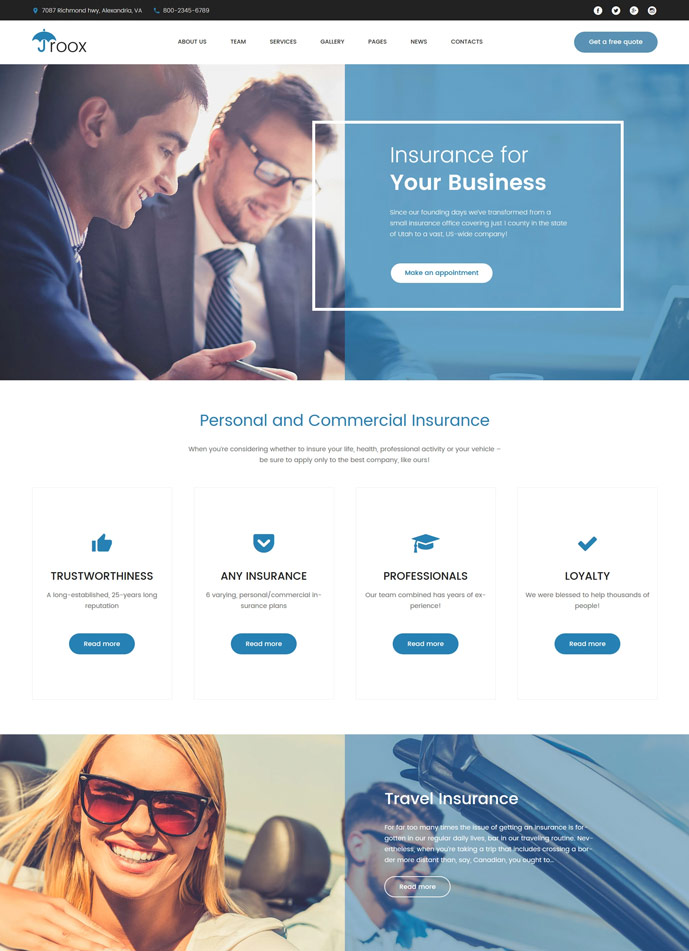The image depicts a vertical computer screen with a predominantly white background. At the top, there is a black navigation bar with the text "JROOX" in the top-left corner. Notably, the letter 'J' is stylized as a blue umbrella. Several tabs are positioned across this top bar, along with a circular, rectangular button.

On the left side of the screen, there is a large picture featuring two men who are smiling and laughing, seemingly engaged in a discussion while looking down at some paperwork. To the right of this image, the picture transitions into a large, blue square, which is semi-transparent and blurred. Overlaying this blue square is a white box containing the text "Insurance for your business," followed by some smaller print and a white circular button.

Below this main section, the caption "Personal and Commercial Insurance" appears in blue text. Beneath this caption, four icons are aligned horizontally across the screen: a thumbs up, a small down arrow, a graduation cap, and a check mark, each accompanied by text descriptions.

At the bottom of the screen, there is another rectangular segment. On the left side of this section, an image of a girl wearing sunglasses and smiling is displayed. On the right side, the text "Travel Insurance" is presented against a similar blue and white background.